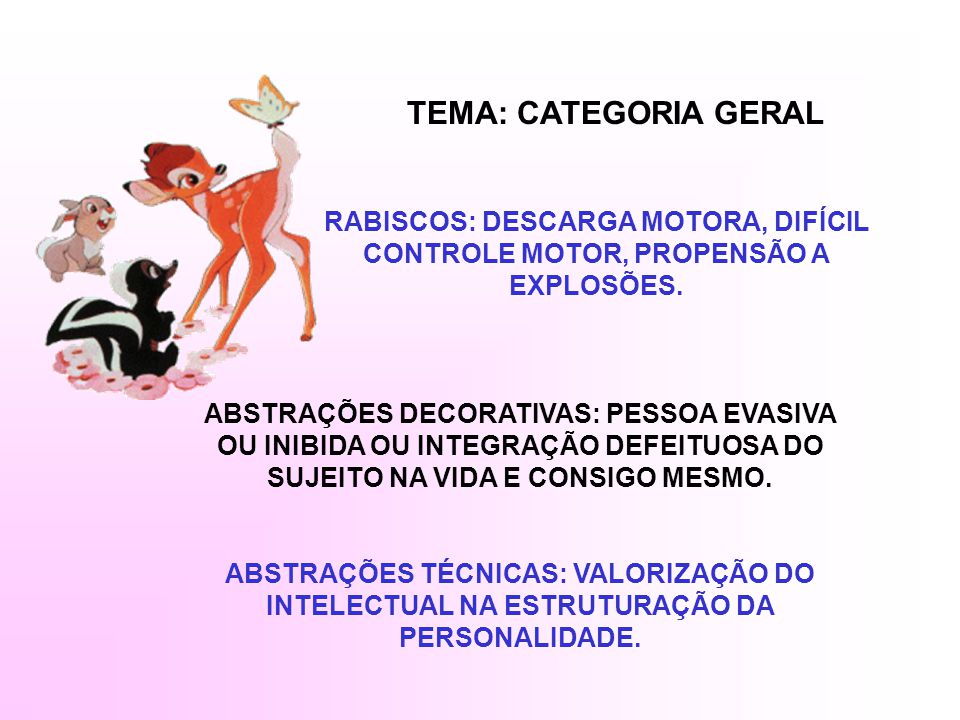The image appears to be a presentation slide, possibly from a classroom setting or another educational context. In the upper left corner, there's a colorful illustration featuring several Disney characters: Bambi, adorned in orange hues, gazes at a white and orange butterfly perched on her tail. Below Bambi, a black and white skunk is depicted, and to the left, a light brown rabbit can be seen. The ground beneath these characters is scattered with white and pink flower petals, which appear to be digitally added. The rest of the slide is dominated by text in what seems to be Spanish, with black and blue fonts. The text includes phrases such as "tema: categoria general" and "rabisco: descarga motora dificil, controle motor, propensao a explosoes." The image lacks a detailed background, focusing instead on the characters and textual elements. The predominant colors include white, pink, purple, black, various shades of brown, orange, and blue, all set against a white background.